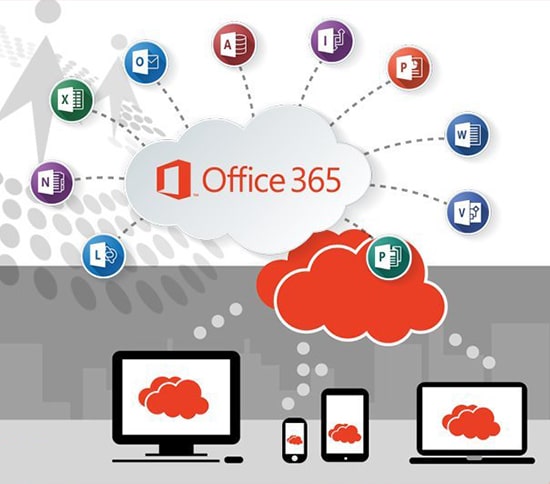The image provides a visual representation of the Office 365 application suite. Dominating the center of the image is a large white cloud bearing the text "Office 365" written in bold orange letters. 

Radiating from this central cloud, several dashed lines stretch outward, each culminating in a circle that encloses the icons of various Office 365 applications. Notable among these are Microsoft Excel, Outlook, Word, Visio, PowerPoint, and Access, along with other recognizable yet unspecified tools.

Below the central white cloud, two smaller orange clouds are featured. These orange clouds also have dashed lines extending from them, connecting to symbols that represent different types of hardware: a desktop computer, a smartphone, a tablet, and a laptop. Each of these connected devices displays the same orange cloud, symbolizing the use of Office 365 applications across multiple platforms.

The background is bifurcated, with the upper portion in white and the lower in gray, providing a clean yet contrasting backdrop that highlights the cloud and device icons. This image effectively communicates that Office 365 is a cloud-based service offering multiple applications accessible across various devices.